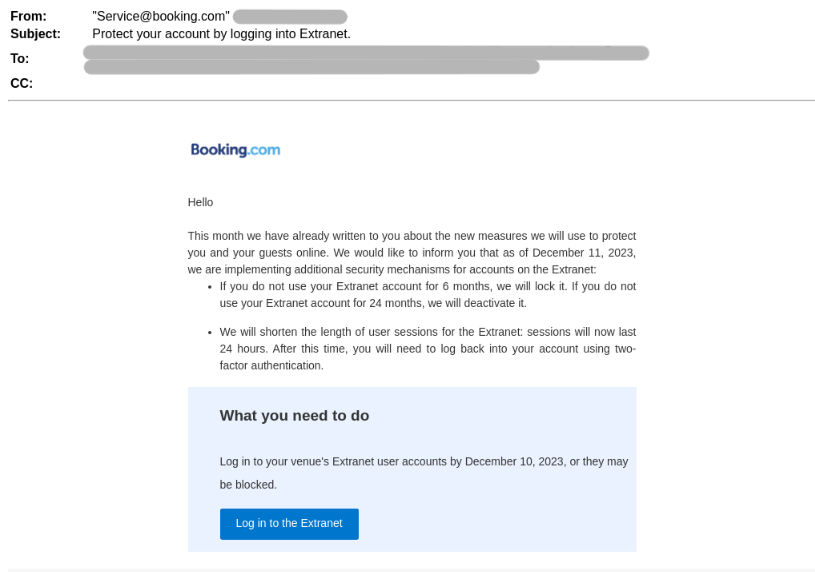**Descriptive Caption for the Email Image:**

The image depicted is a screenshot of an email from Booking.com, which appears on a white background provided by the computer screen. The email interface suggests access via email applications on a computer or smart device. 

At the top, the email metadata section is visible. On the left-hand side, labels such as "From," "Subject," "To," and "Cc" are bolded. Opposite "From," the sender is identified as "service@booking.com," with adjacent content that is grayed out. The "Subject" line reads "Protect your account by logging into Extranet." The recipient's address under "To" is entirely grayed out, and beneath it lies another gray line. The "Cc" field is empty. A thin black line separates this metadata from the main body of the email.

In the content section, the sender, Booking.com, greets the recipient formally, starting with "Hello." The email outlines new security measures for user accounts on the Extranet, effective December 11, 2023. It mentions prior communication regarding these changes to protect the account holders and their guests. Key points include:

- Inactivity for six months will result in account lockout.
- Inactivity for 24 months will lead to account deactivation.
- User session times will be shortened to 24 hours, necessitating re-login through two-factor authentication thereafter.

A blue box titled "What you need to do" in bold stands out, urging users to log into their Extranet accounts by December 10, 2023, to avoid potential blockage. It ends with a darker blue button displaying "Log into Extranet" in white text, providing a clear call to action for recipients.